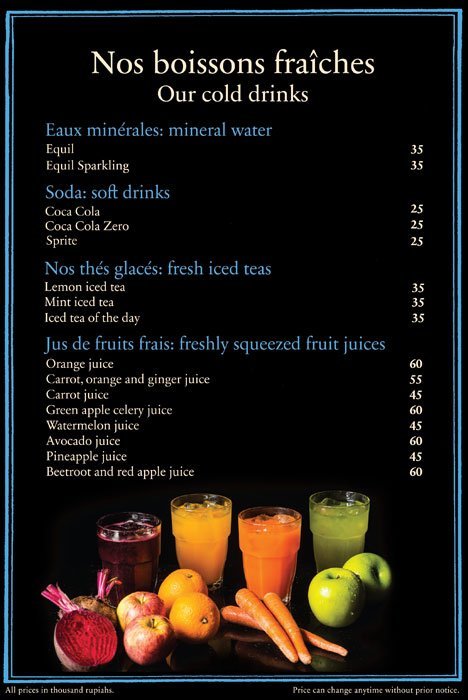The image is a detailed menu displayed on a black background, with the top half dedicated to various categories of beverages and their respective prices, written in both English and another language. At the top of the menu, "Cold Drinks" is prominently displayed in white font. The menu includes sections for "Minimal Water" highlighted in blue, offering multiple options and their prices, along with listings for soft drinks like Coca-Cola, Coca-Cola Zero, and Sprite. Below these, there is a section for fresh iced teas, detailing different types and their prices, followed by another section for freshly squeezed fruit juices including orange, carrot, and apple juices.

The bottom half of the menu features images of several fresh fruits and corresponding pressed juices, which appear as props to illustrate the freshness of the offerings. Visually, there are green apples in front of what seems to be apple juice, carrots with carrot juice, and additional fruits like pears and beets accompanied by their respective juices in shades of red, yellow-orange, dark orange, and clear lime green. Each juice is presented in a glass, from left to right, in the described order. The text at the bottom reads "NOS Boysen's Freshest Alcohol Drinks," followed by further listings, reinforcing the freshness and natural quality of the beverages offered.